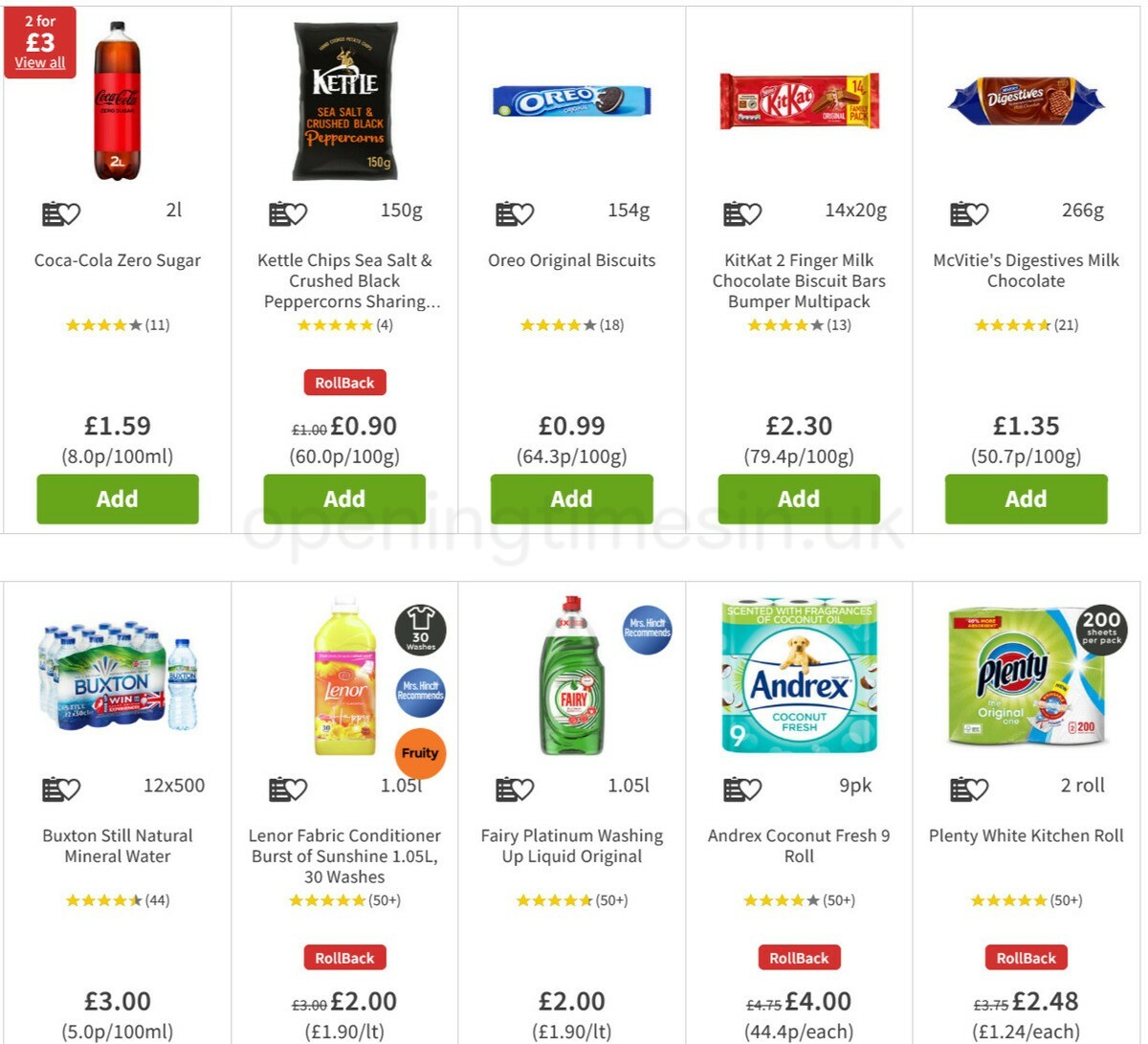The image depicts a website interface of a retail or grocery store. The web page is organized into two rows and five columns. Each item listed has an adjacent "Add" button to add the product to the cart. 

In the first row, the items displayed are:
1. Coca-Cola Zero, priced at £1.50.
2. Kettle Chips Sea Salt and Crushed Black Peppercorn (sharing size), in a black bag, priced at £0.90 and marked as a "Rollback" deal.
3. Oreo Original Biscuits, priced at £0.99.
4. KitKat Two-Finger Milk Chocolate Biscuit Bars (bumper multi-pack), priced at £2.30.
5. McVitie's Digestive Milk Chocolate Biscuits, priced at £1.35 and also labeled as a "Rollback" deal.

In the second row, the items listed are:
1. Buxton Natural Mineral Water, priced at £3.00.
2. Lenore Fabric Conditioner, priced at £2.00 and marked as a "Rollback" deal.
3. Fairy Platinum Dishwasher Tablets, priced at £2.00.
4. Andrex Coconut Fresh Toilet Paper (9 pack), priced at £4.00 and marked as a "Rollback" deal.
5. Plenty Kitchen Roll, priced at £2.48 and marked as a "Rollback" deal.

The "Rollback" deals are prominently highlighted in red, making the discounted items easily identifiable for shoppers.